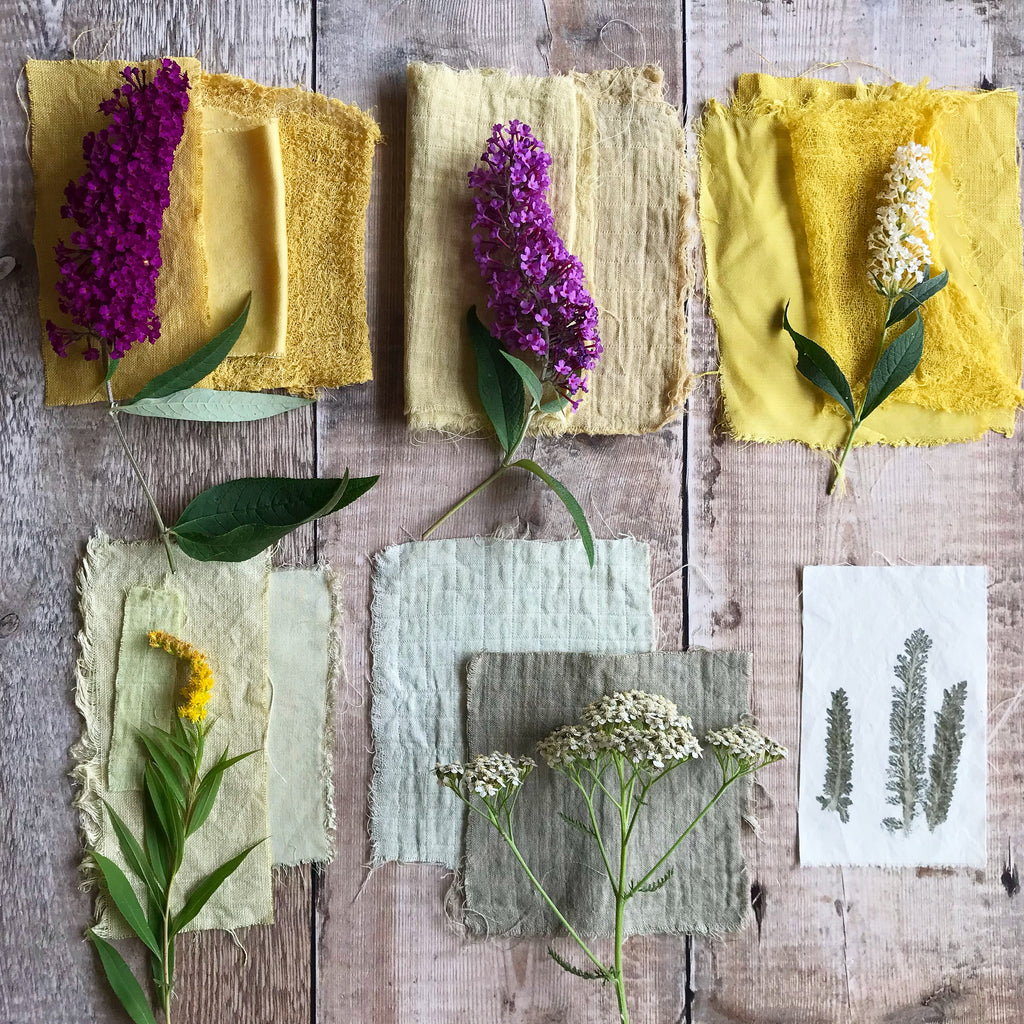The image is a professionally taken, brightly lit but subtly shadowed tableau of dried flowers meticulously arranged on a white oak wooden floor. Each of the six patches of fabric beneath the flowers contrasts beautifully with the plants lying atop them, enhancing their vibrant colors and intricate details. 

In the top row, from left to right, there are two purple flowers: the leftmost has a thin stem and large dark green leaves, lying on a yellow cloth. Next to it, a lighter purple, almost violet flower with a thin stem and lighter green leaves, also rests on a yellow cloth. On the right, a cone-shaped white flower with dark green foliage sits on a lighter yellow fabric.

In the bottom row, to the left, a long-stemmed yellow flower with closely spaced dark green leaves is placed on an olive green cloth. Adjacent to it, a broccoli-like white flower with creamy beige hues and darker green stems sits on a gray cloth layered over a light blue one. Finally, to the right, thin, dark green plant pieces are laid out on a pristine white cloth. This artistic composition, with its array of colors and textures, likely showcases the flowers in preparation for drying.